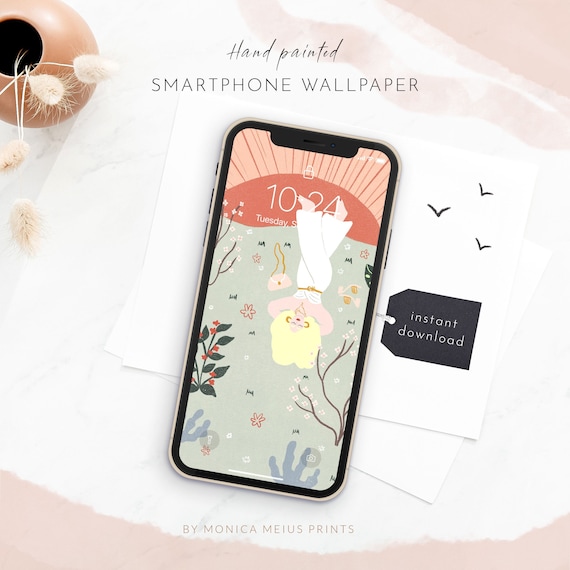The image is a full-color, vertical rectangular advertisement with a beige and white background. It features an assortment of elements arranged on a surface. In the top left corner, there is a rust-colored flower pot with white flowers and a cylindrical vase containing dried reed-like flowers for an artistic touch. The centerpiece of the image is an iPhone, displaying a hand-painted smartphone wallpaper that shows a red sun rising over a field with a woman laying in it, wearing a white jumpsuit with large blonde hair. Beside the phone is a small parcel tag labeled "instant download". Above the iPhone, in calligraphy and typed text, it reads "hand-painted smartphone wallpaper", accompanied by three small, bird-like ticks. At the bottom, the advertisement credits "by Monica Mayes Prince" in light grey font. The entire scene appears to be set on a granite countertop, giving it an earthy and sophisticated feel.